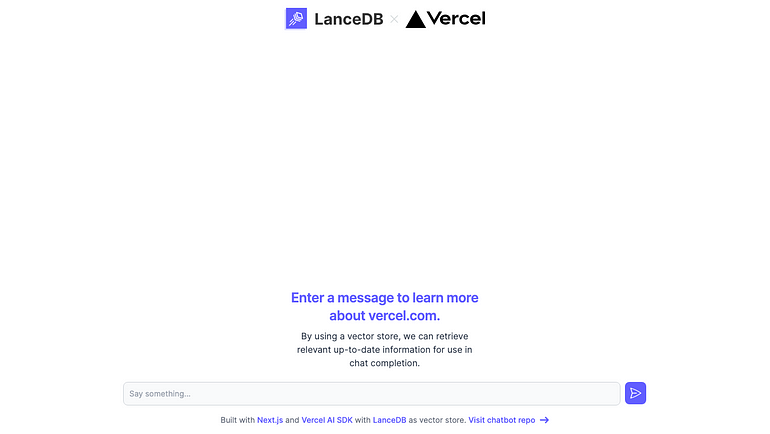Here is the cleaned-up and detailed caption:

"A screenshot from a website or app's interface features a minimalist design with prominent use of purple and white. At the top left corner, a white logo sits within a purple square next to the black text "Lance D.B." Appearing after is a black triangle followed by the text "Vercell". The central part of the screenshot is largely a white background. Near the bottom, purple text prompts users to 'Enter a message to learn more about Vercell.com'. Below, black text reads, 'By using a vector store we can retrieve relevant up-to-date information for use in chat completion'. A text input bar labeled 'Say something' is visible further down. To the right of this bar is a purple square featuring the 'CEND' logo. Below, in gray text, it reads, 'Built with Next.js and Vercell AISDK with Lance D.B. as a vector store. Visit chatbot repo,' accompanied by a right-pointing purple arrow."